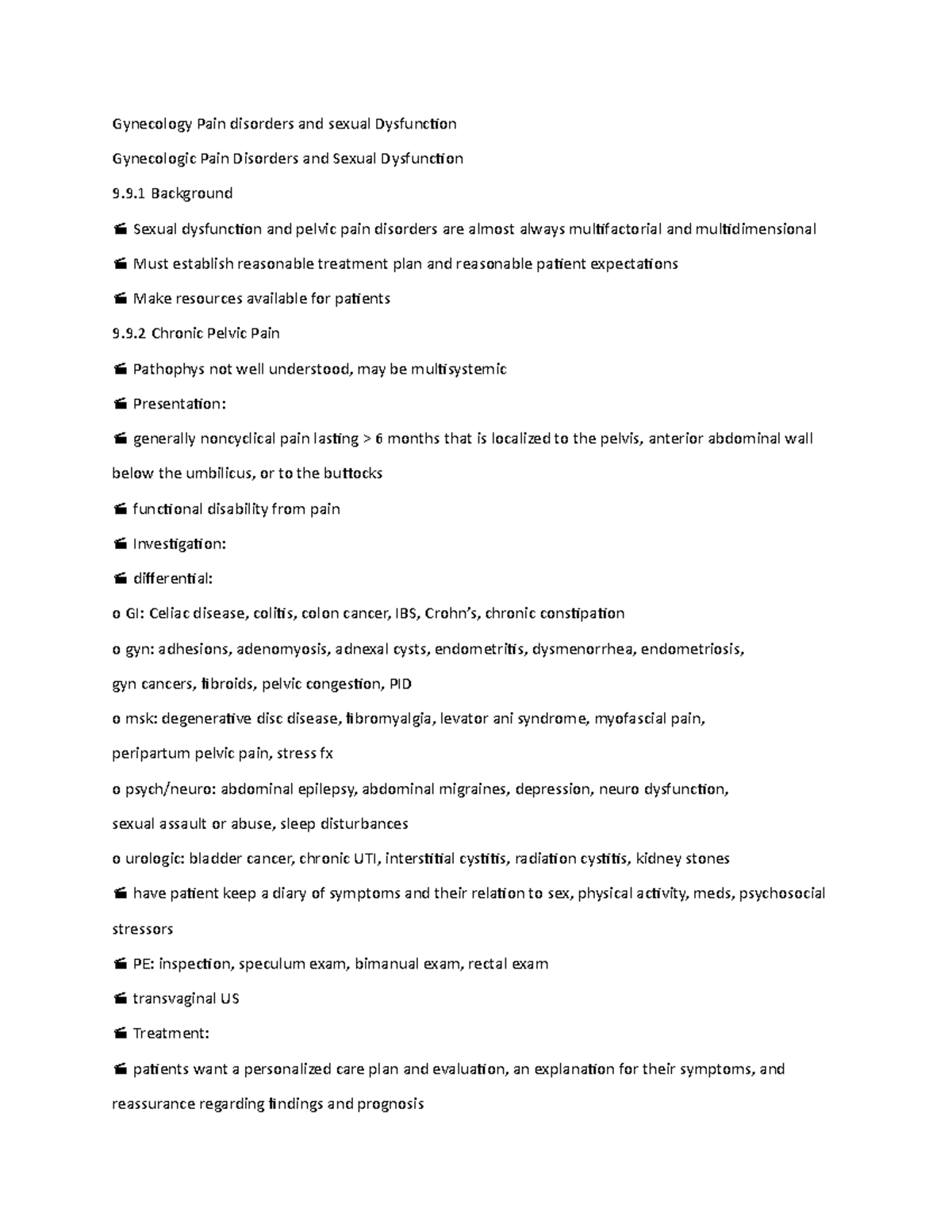**Detailed Descriptive Caption:**

The image is an informative poster detailing the complexities and treatment considerations for gynecological pain disorders and sexual dysfunction. The top section prominently displays the topics "Gynecology, Pain Disorders, and Sexual Dysfunction," followed by a reiteration of these subjects. It outlines the background with a director's icon, stating, "Sexual dysfunction and pelvic pain disorders are almost always multifactorial and multidimensional." 

Next, it stresses the need to "establish a reasonable treatment plan and reasonable patient expectations," accompanied by another director's icon. Another point highlighted with the same icon is to "make resources available for patients."

The poster then focuses on chronic pelvic pain, denoted as section 9.9.2. This section, introduced with a director's icon, notes, "Pathophysiology is not well understood, maybe multisystematic." The presentation, underscored again by a director's icon, indicates "generally nonspecific pain lasting less than six months," which is localized to the pelvis, anterior abdominal wall, below the umbilicus, or the buttocks.

Furthermore, there's a mention of an investigation section labeled as "differential," which includes a detailed list of potential diagnoses such as celiac disease, colitis, colon cancer, IBS, Crohn’s disease, chronic constipation, gynecological issues like adhesions, adenomyosis, endometriosis, and dysmenorrhea.

The poster emphasizes the need for "functional disability from pain" and notes that "patients want a personalized care plan, an evaluation, an explanation for their symptoms, and reassurances regarding findings and prognosis." The entire content is presented on a white background with black text, and various segments are highlighted with director-style icons, reminiscent of movie industry clapperboards, adding a visual cue to the informational layout.